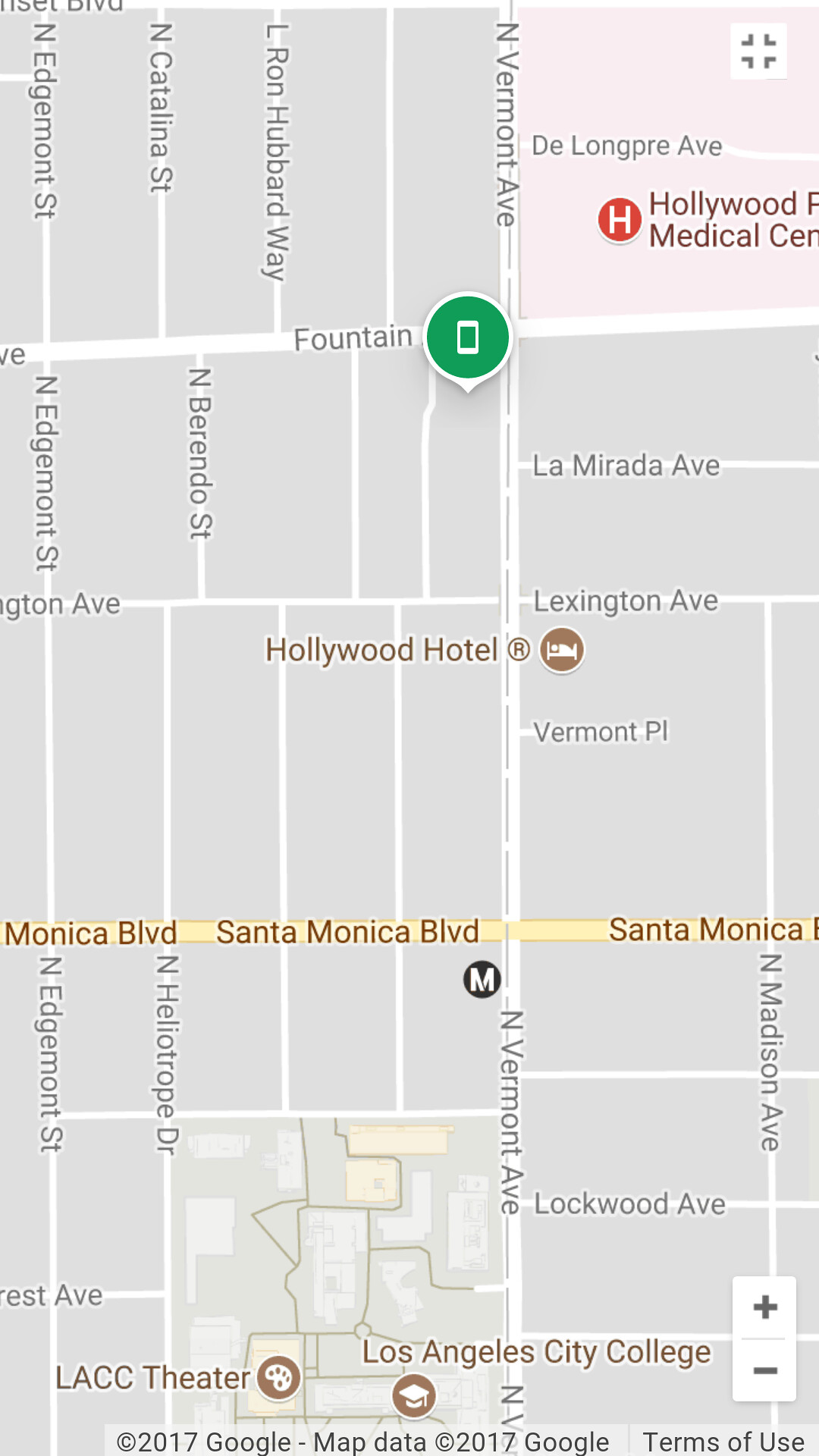An image of a Google Maps screenshot displaying a detailed section of Los Angeles, with a focus on the area around Santa Monica Boulevard. The map is in a light gray color palette, with roads highlighted in white. Prominent roads are depicted as slightly wider lines, providing clear visibility of major routes. Santa Monica Boulevard is depicted in a beige color, signifying its importance.

Notable landmarks and streets mentioned include the Hollywood Medical Center in the top right, highlighted by a pink area. A small green bubble with a phone icon suggests the presence of cell phone activity in the vicinity. Key streets such as Fountain Avenue, Lockwood Avenue, Helicopter Drive, Edgemont Street, Madison Avenue, North Vermont Avenue, and Lexington Avenue are visible.

Additionally, landmarks like Los Angeles City College, LACC Theater, the Hollywood Hotel, La Mirada Avenue, and L. Ron Hubbard Way are marked on the map, offering a comprehensive view of this section of Los Angeles. The bottom of the map credits "2017 Google Maps data" and includes terms of use.